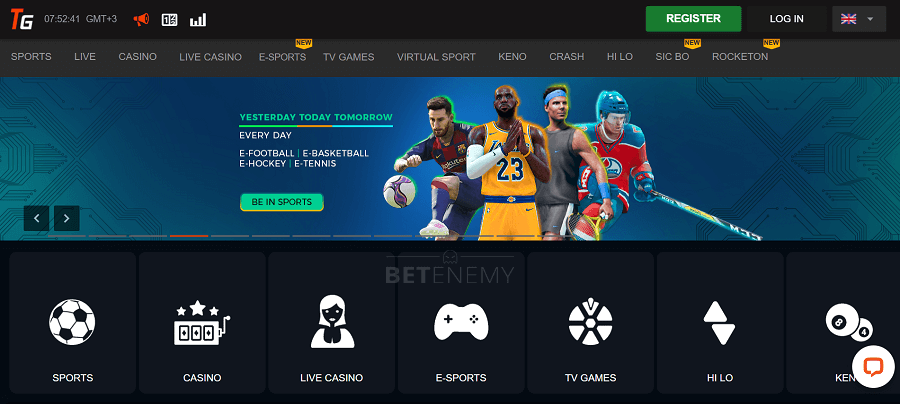**Caption:**

The screenshot showcases a website with the initials "TG." In the upper left corner, a prominent red "T" and a white "G" logo stands out against the primarily black and dark gray background of the site. Dominating the top part of the page is a large rectangular image featuring a dark blue and dark green gradient, with well-known professional athletes at its center. Among them are LeBron James and Rafael Nadal, accompanied by an unidentified hockey player and soccer player. Superimposed over the players is text reading "Yesterday, Today, Tomorrow" followed by "Every Day." Additional labels within the image include "eFootball, eBasketball, eHockey, eTennis," and a green button labeled "Be in Sports." 

Below this visual section, the website features several clickable buttons or sections, offering categories such as Sports, Casino, Live Casino, eSports, TV Games, and High Low. The overall design and arrangement suggest a dynamic, sports-focused theme with interactive gaming options.